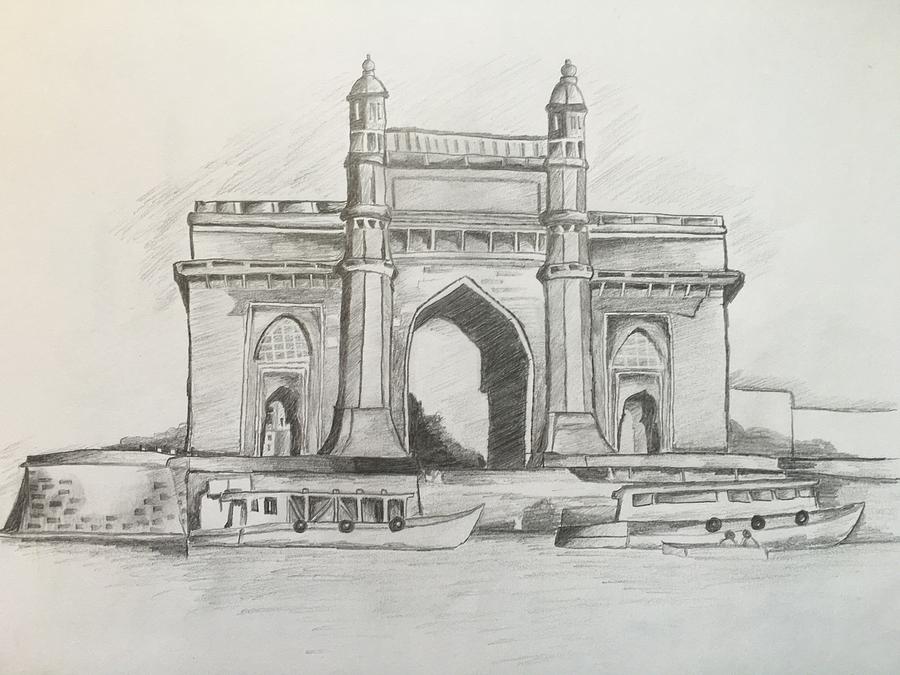The image is a detailed pencil sketch depicting a tranquil waterway bordered by gently bobbing boats resting against the shoreline. Though no piers or docks are explicitly visible, the scene suggests a pier-like atmosphere. In the background, a tall, stately building towers over the water with regal prominence. The structure boasts a couple of turrets and a significant arched gateway, which is shadowed to convey depth and grandeur. This large, open gateway, seemingly capable of accommodating large entities, is flanked by arched windows, adding to the building's imposing character. The sketch artist has meticulously used shading to add texture and dimension to both the building and the sky. The scene is devoid of human figures, focusing entirely on the magnificent architecture and serene waterway.